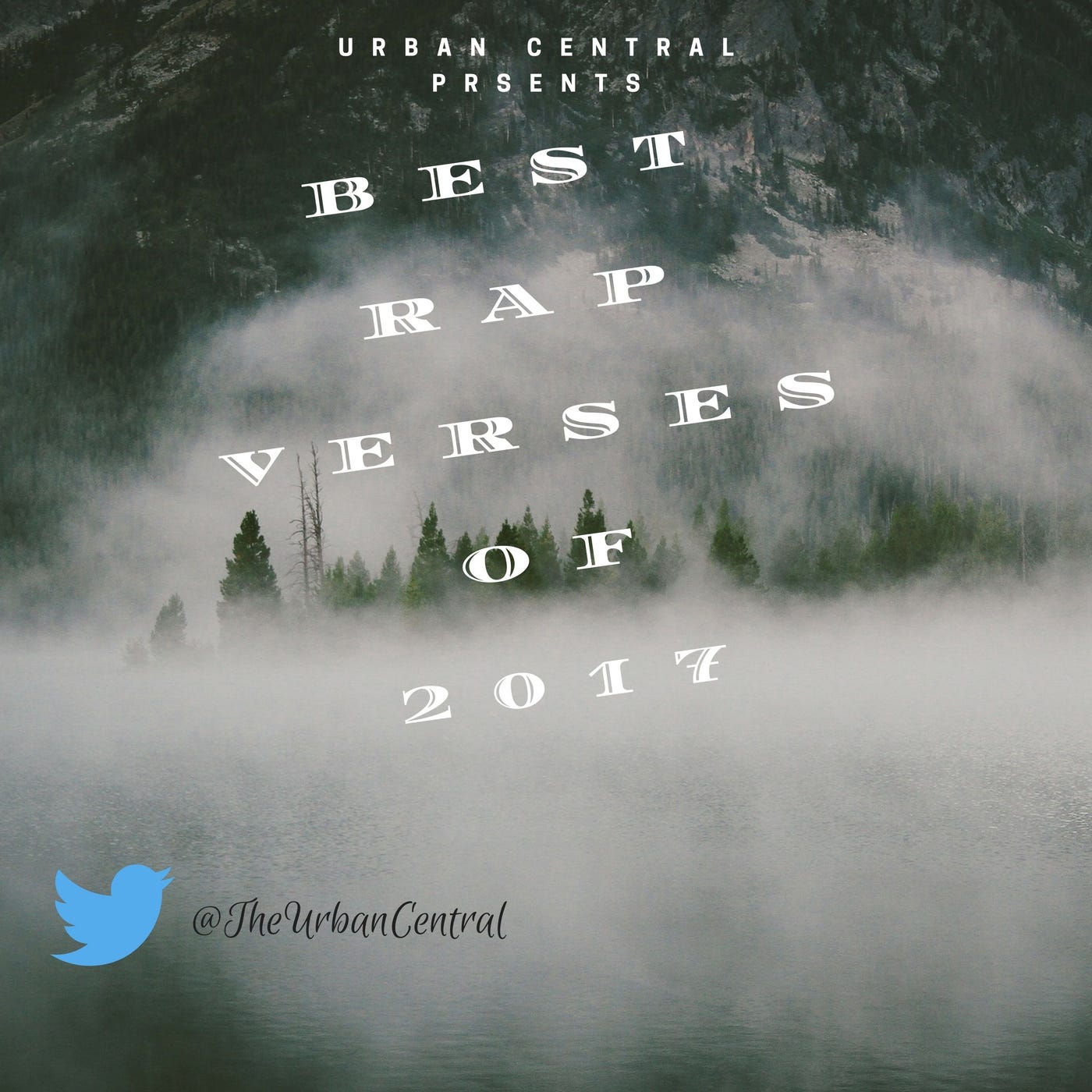This square poster-style image features a top-down view of a mountainous landscape, predominantly in subdued gray, black, and white tones, with a hint of dark and light green creating a cold, almost monotone atmosphere. The rocky mountains and trees are partially shrouded in a thick, hazy white fog that adds an element of mystery and depth to the scene. Overlaying this foggy, forested background, the text "Urban Central Presents Best Rap Verses of 2017" is prominently displayed in bold, uppercase white letters across the top. The title is crafted in a formal font, while "Best Rap Verses of 2017" shifts to a more playful, slightly slanted style, maintaining the all-caps presentation. At the bottom left of the image, the blue Twitter bird icon is clearly visible, followed by the handle "@theurbancentral" in a small, black font. The overall design is minimalistic yet striking, effectively capturing attention with its blend of text and natural, foggy scenery.